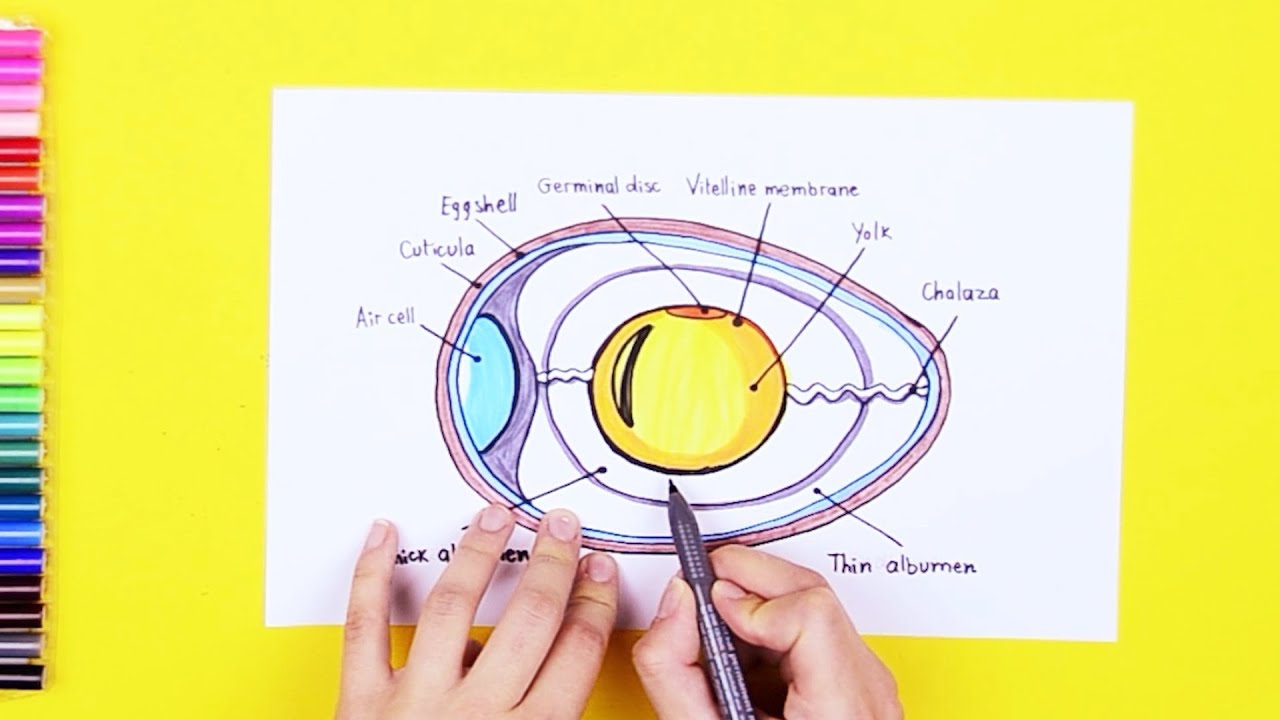An image designed for a science or art blog features a detailed, hand-drawn diagram of an egg's anatomy on a white piece of paper, placed on an unnaturally bright yellow desktop, possibly photoshopped. The image is in landscape layout with colorful marker caps lined up along the left side, displaying a spectrum from shades of fuchsia to pink, red, purple, blue, green, and black. In the center of the paper, a large oval cross-section of an egg is meticulously colored with pinks, blues, purples, yellows, and oranges, and segmented with black lines that label each part. Two Caucasian hands are at the bottom of the image; the left hand pressing on the paper and the right holding a pencil, indicating active drawing. The egg diagram comprises labels such as the pink outer eggshell, a blue inner membrane, the centrally located yolk, and structures such as the air cell, Vitelline membrane, chalaza, germinal disk, and thin albumen. This vivid, informative illustration emphasizes both creativity and scientific detail, making it suitable for educational purposes in either a science or art context.